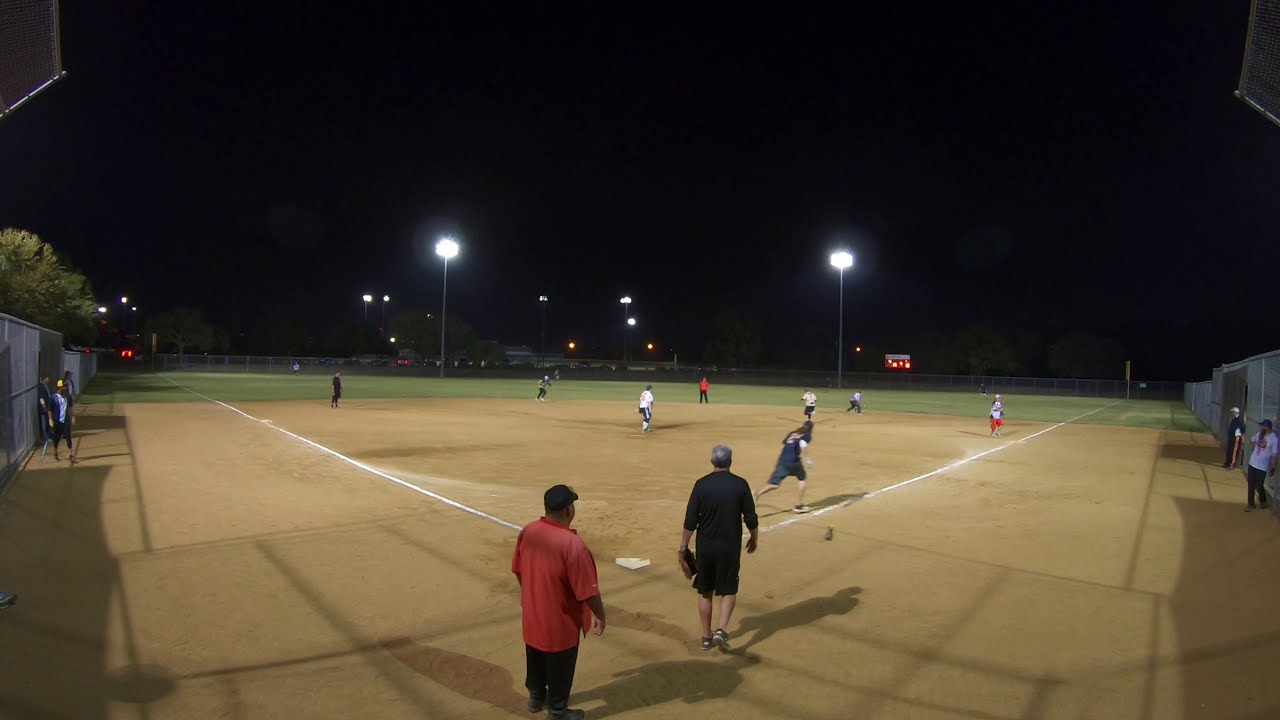This is a detailed photograph of an evening baseball game, clearly taken at night under a dark sky illuminated by bright white stadium lights at the edges of an outdoor field. The view is from behind the home plate, showing the perspective of the umpire, who is wearing a red short-sleeved T-shirt and black pants, without any official equipment, indicative of an informal game. The catcher, dressed in a black long-sleeved T-shirt and black shorts, along with the umpire, is looking towards the right where the ball has presumably gone. A runner, identifiable by his blue attire and forearm guard with a visible number on his shirt, is sprinting towards first base. In the background, chain link fences flank both sides of the field, with additional details like trees, lights, and a scoreboard under the right floodlight. The field itself is neatly divided with a sandy infield and a grassy outfield, emphasizing the game's setting under the night sky.